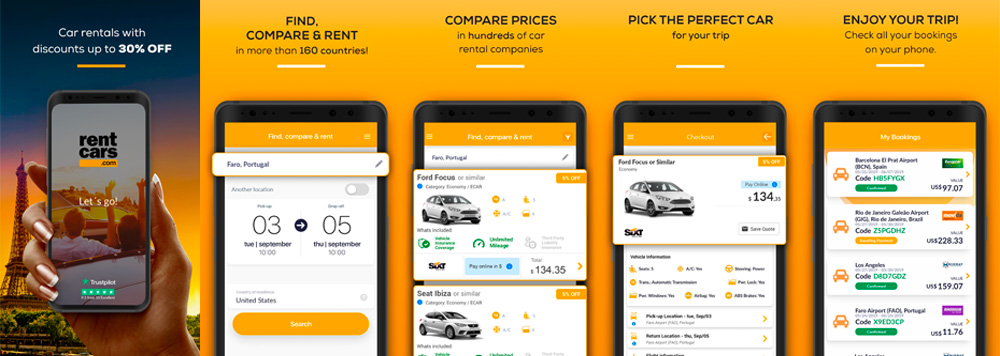In this vibrant promotional screenshot, the primary backdrop is a vivid orange color. On the left side of the image, there is a gray cell phone being held by a female hand with gold nail polish, emerging from the lower right corner. The screen of the phone displays a captivating message: "Rent cars, let's go. Car rentals with discounts up to 30% off."

To the right of this main section, the orange background frames four additional images of cell phones, aligned horizontally. Each phone screen showcases a different step in the car rental process:

1. The first phone screen reads: "Find, compare, and rent in more than 160 countries."
2. The second phone screen states: "Compare prices in hundreds of car rental companies."
3. The third phone screen advises: "Pick the perfect car for your trip," featuring an image of a white Ford Focus sedan available for $134.
4. The fourth phone screen announces: "Enjoy your trip. Check all your bookings on your phone," illustrating this with a "My Bookings" screen.

This detailed layout serves as a step-by-step guide for users looking to rent cars conveniently with substantial discounts.